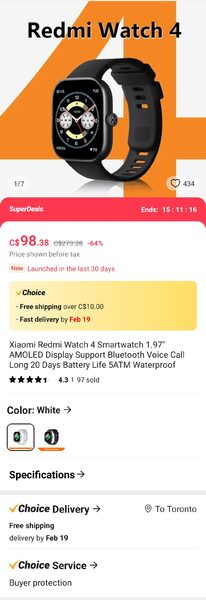The image features a prominent promotional display for a Black Xiaomi Redmi Watch. The layout of the advertisement includes various elements, arranged as follows:

1. At the top center, in black text, it reads "Redmi and Redmi Watch 4".
2. The background is predominantly white, with a large orange numeral "4" in the background, occupying much of the space.
3. In the foreground is the Black Xiaomi Redmi Watch, featuring a black band.
4. Towards the bottom left, the text reads "1/7", while on the right it shows "434 likes".
5. Below this, a red band with white text highlights, "Super Deals".
6. On the right side of this band, there's an expiration notice: "Ends 15/11/16".
7. Just below, a price section lists "$98.38 CAD" in red font on a white background. The original price of "$279.20 CAD" is visibly crossed out, indicating a 64% discount.
8. Additional information includes: "Price shown before tax", "New launched in the last 30 days", "Choice Free shipping over $1 CAD", and "Fast delivery by February 19th".
9. At the bottom, accurate product details are given: "Xiaomi Redmi Watch 4 Smart Watch", "1.97 AMOLED display", "Supports Bluetooth voice call", "Long 20-day battery life", and "5ATM waterproof".

This detailed and enticing layout aims to attract potential buyers with its clear information and notable discounts.